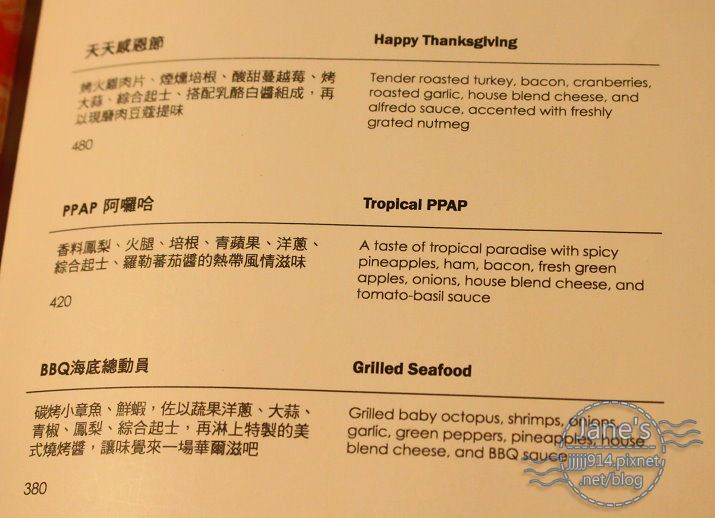The image is of a menu printed on cardstock, featuring both Chinese characters on the left and their English translations on the right, centered directly in the image. The menu is in black font with an off-white background and includes dishes such as: "Happy Thanksgiving" - tender roasted turkey, bacon, cranberries, roasted garlic, house blend cheese, and alfredo sauce, accented with freshly grated nutmeg; "Tropical Ppap" - a taste of tropical paradise with spicy pineapples, ham, bacon, fresh green apples, onions, house blend cheese, and tomato basil sauce; and "Grilled Seafood" - grilled baby octopus, shrimps, onions, garlic, green peppers, pineapples, house blend cheese, and barbecue sauce. The color palette includes light blue, brown, and red. In the bottom right corner, there's a watermark that reads "jamesjjjj914.pixnet.net/blog."